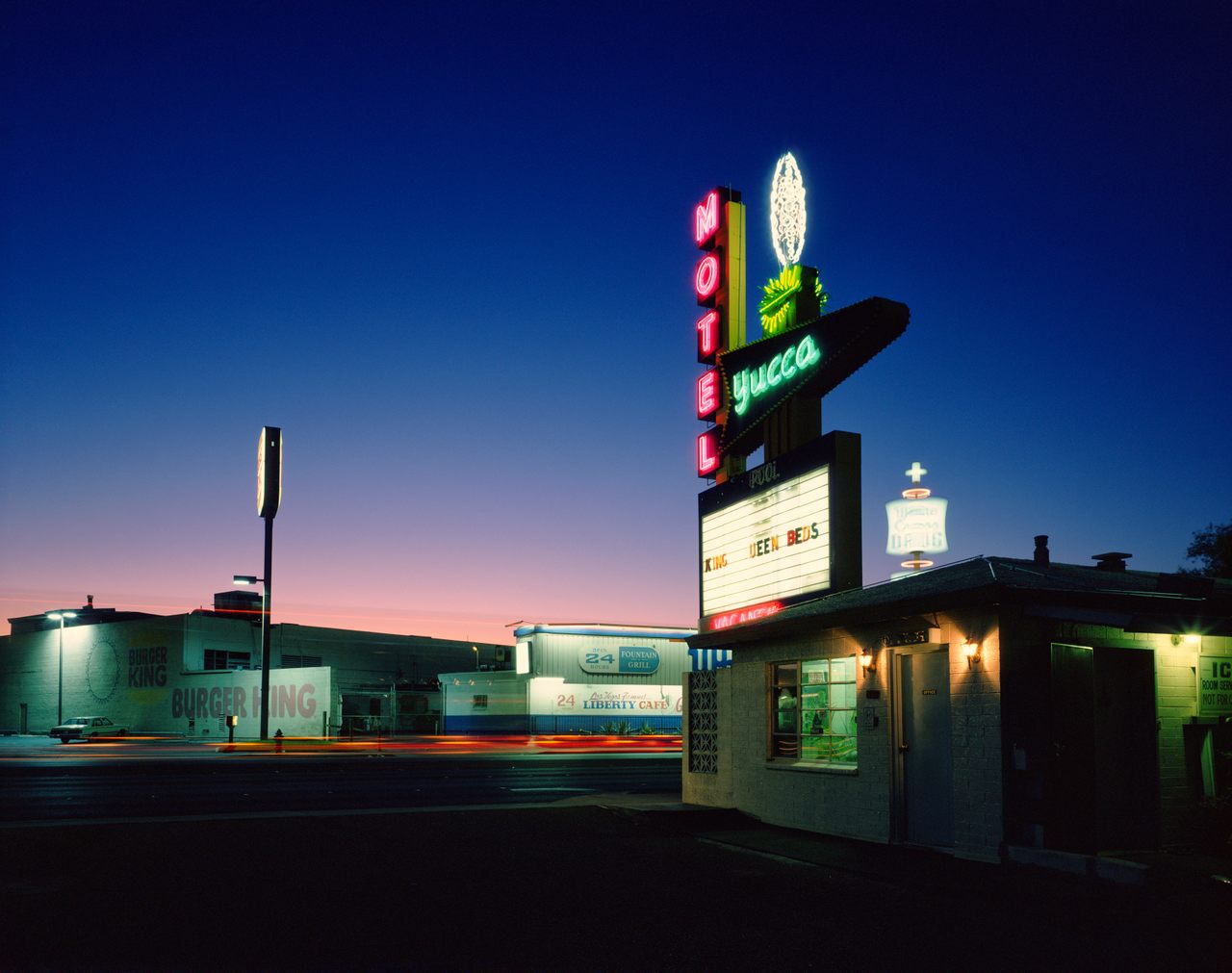The image depicts a small town city street at dusk, transitioning from a dark blue to a pink sky. Dominating the right side is the Yucca Motel, featuring a prominent vertical neon red sign that vertically spells out "Motel," paralleled horizontally at the base by "Yucca" in vibrant green neon. Atop the neon letters, a depiction of a Yucca plant is visible, extending over the "M" in "Motel,” with an additional oval-shaped bulb. Beneath the green "Yucca" sign, a multi-colored neon sign reads "King Queen Beds," although the "Q" in "Queen" is missing. Further below, the text states "Air Conditioned Units." The motel building itself is constructed of white brick, accentuated by a blue door and a window, through which the office interior is faintly visible but without discernible details.

Across the street, to the lower left, stands a white brick building with the Burger King logo and the name "Burger King" displayed in large red letters. Adjacent to this building is a 24-hour Liberty Cafe. A neon sign indicating "Burger King" is also present in front of the establishment. The scene is set against the backdrop of twilight, capturing the small town's serene yet lively ambiance.